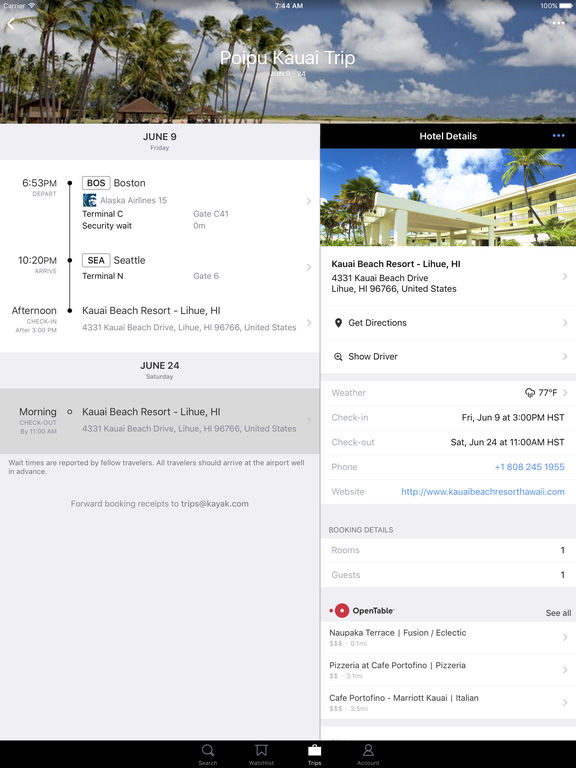Screenshot of a travel itinerary on a tablet displaying details from the travel website "Poipukauaitrip," taken at 7:44 AM. The tablet shows full mobile data coverage and a 100% battery life, although it is not currently charging.

Visible travel details include a booked flight departing from Boston at 5:53 PM and arriving in Seattle at 10:20 PM. It’s unclear if the arrival time accounts for time zone differences. Following the flight leg, the itinerary details accommodations at the Kauai Beach Resort in Lihue, Hawaii, located at 4331 Kauai Beach Drive, Lihue, Hawaii, 96766, United States. The guest is set to check in on Friday, June 9th, and check out on Saturday, June 24th, with the precise check-out time listed as 11:00 AM.

The resort information includes options for directions, showing a driver, and current local weather conditions (77°F). Also included are the hotel's phone number, website, and booking details. Restaurant reservations through OpenTable are noted, featuring three dining options: The Terrace, offering fusion and eclectic cuisine; Pizzeria at Cafe Portofino; and Marriott's own Italian restaurant, Cafe Portofino.